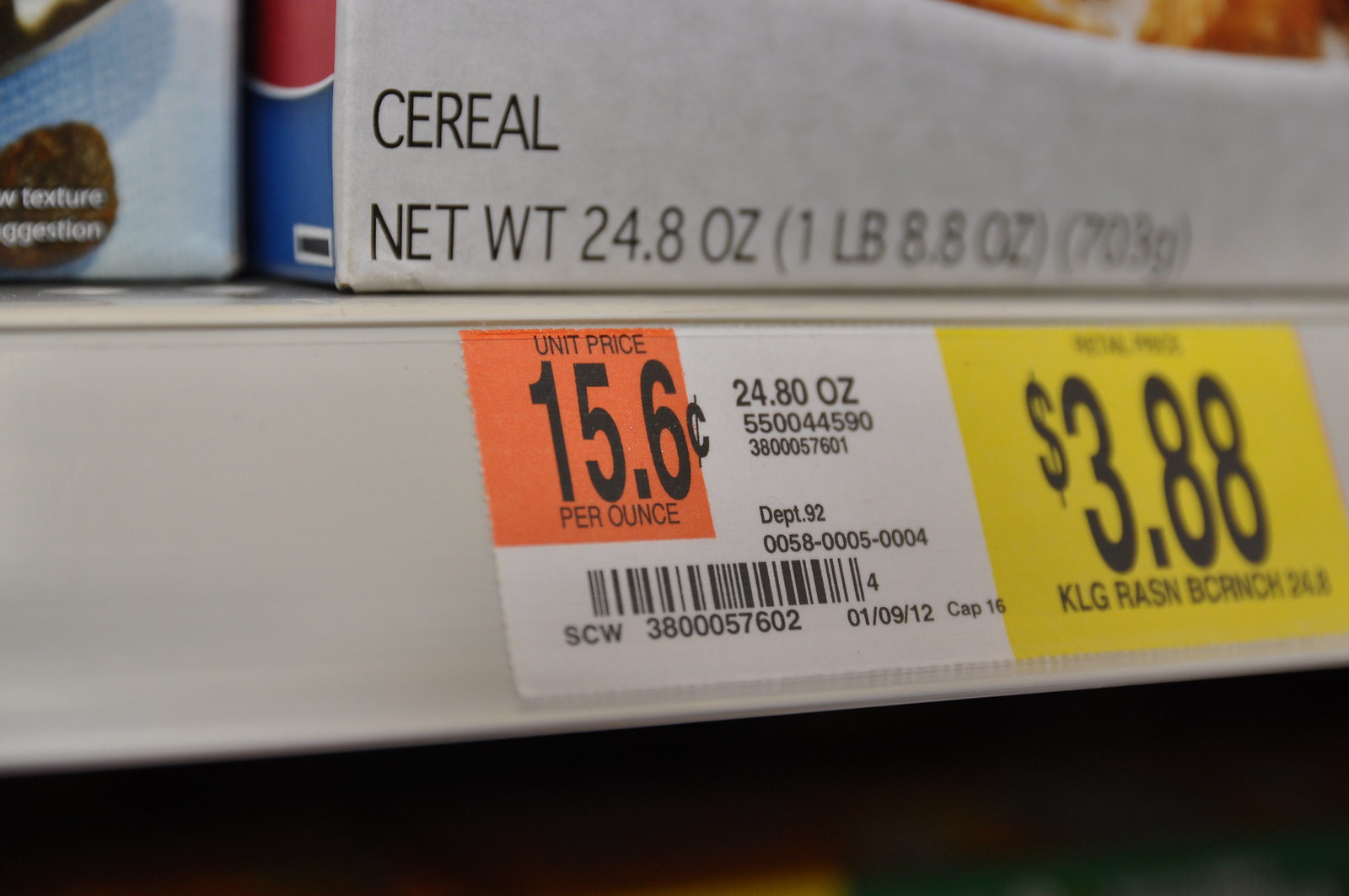In the cereal aisle of the grocery store, a price sticker for Kellogg's Raisin Bran Crunch is prominently displayed on the shelf. The price is marked in bold black letters as $3.88, set against a striking red background. To the left of this price, an orange section of the sticker details the unit price, clearly noting it as 15.6 cents per ounce. Situated directly above this sign is a box of cereal with a net weight of 24.8 ounces. Although the specific cereal box isn't fully visible, it is reasonable to deduce that it is indeed Raisin Bran Crunch, given its position above the corresponding price sticker.